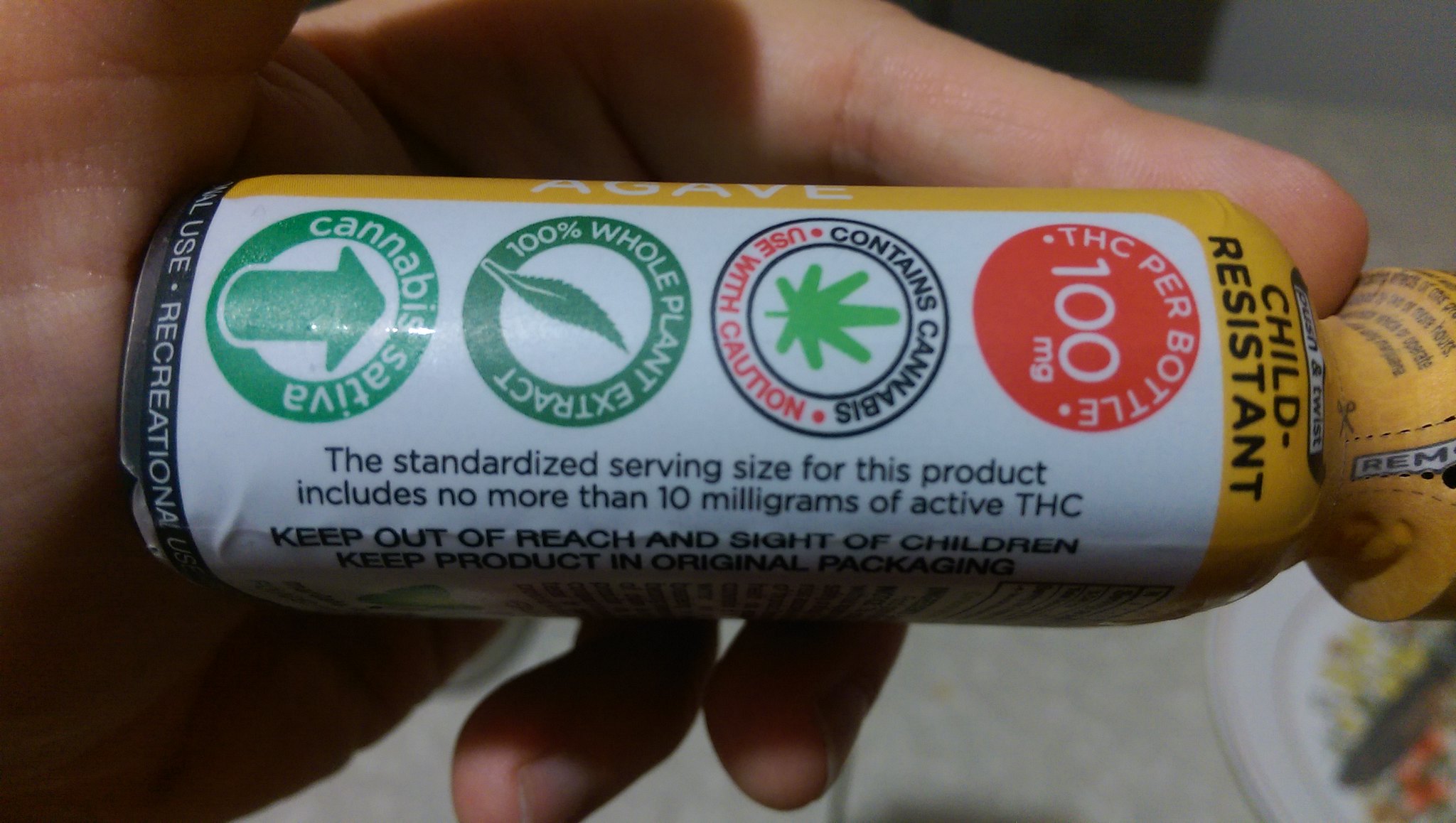In the image, a person's left hand is seen extending into the frame from the left side, with their palm facing inward and their pointer finger resting on top of a cylindrical bottle. The bottle, which appears to be around 4 inches long and 1.5 inches wide, is a cannabis product featuring a yellow perimeter border and a white central label. The label reads "Agave" at the top, with the letters A-G-A-V-E clearly spelled out. Just below this, on the right side, it states "child resistant." The product's cylindrical design includes a thin neck and a yellow top that seems to be circular but is cut off by the edge of the photo. 

Prominently displayed on the label are four logos, each with specific details: one with a green arrow labeled "Cannabis Sativa," another stating "100% whole plant extract," a third logo featuring a marijuana leaf with the warning "Contains cannabis. Use with caution," and a fourth with a red label indicating "THC per bottle 100 mg." 

Additional cautionary notes on the label inform users that the standard serving size is no more than 10 mg of active THC, and it advises to "keep out of reach and sight of children" and to "keep product in original packaging." The product has not been opened as evidenced by the visible perforation sealing it.